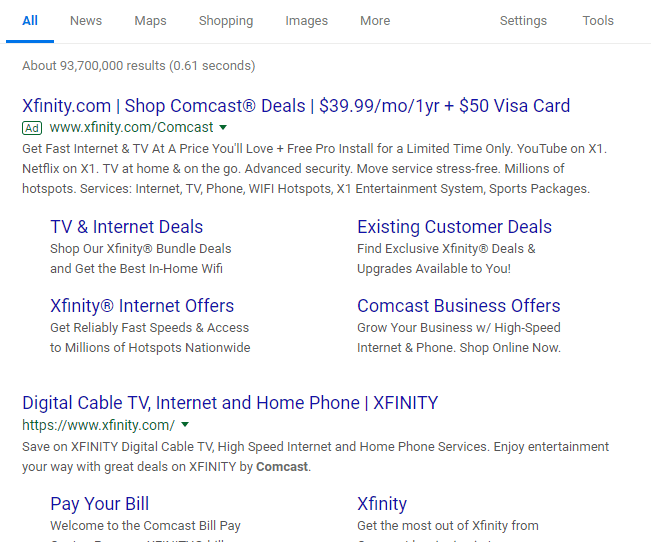A Google search results page is shown in the image. At the top of the page, a horizontal navigation strip lists options such as All, News, Maps, Shopping, Images, More, Settings, and Tools. Most of these options appear in gray, except for the "All" option which is highlighted in blue with a blue underline beneath it. Directly below this navigation strip, the text indicates that there are approximately 93,700,000 search results found in 0.61 seconds.

The very first search result is an advertisement from Xfinity (affinity.com). The ad headlines "Shop Comcast Deals," offering internet and TV services starting at $39.99 per month for one year, plus a $50 Visa card. There is a downward menu indicating additional ad details, including benefits like fast internet, pro installation, YouTube on X1, Netflix on X1, advanced security, stress-free service, and millions of Wi-Fi hotspots.

Below the advertisement, there are two rows of headers, each containing two options. 

The first row features:
1. "Internet and TV Deals": Promotes bundle deals for home Wi-Fi.
2. "Existing Customer Deals": Provides information on exclusive deals and available upgrades for current Xfinity customers.

The second row features:
1. "Xfinity Internet Offers": Highlights fast and reliable internet services.

Each section emphasizes the wide variety of services and features that Xfinity offers to its customers.